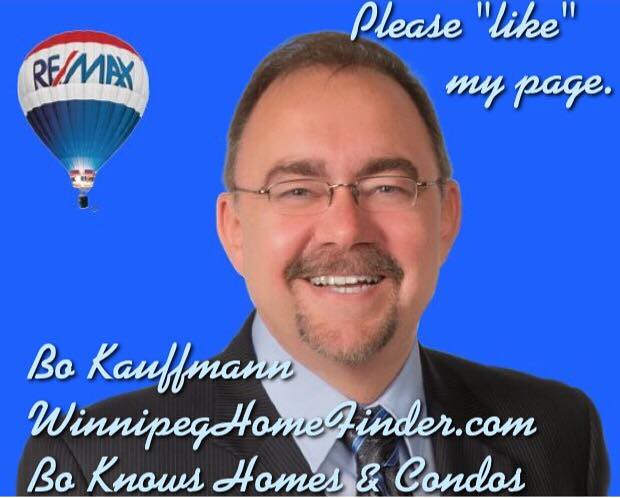This image is a detailed, close-up social media advertisement for a real estate agent. The background is a solid light blue, with a distinctive RE/MAX hot air balloon logo in the top left corner. The balloon is colored in red, white, and blue, with the word "RE/MAX" prominently displayed in large, blue slanted text across the balloon. 

On the right-hand side, the ad features the phrase "Please LIKE my page" in a cursive white font. Dominating the foreground of the image is a middle-aged Caucasian man, estimated to be 40-50 years old. He has short brown hair with a slight receding hairline, blue eyes, and wears glasses. He is smiling warmly and sports a goatee. He is dressed in a dark gray, almost black, pinstriped suit, paired with a light blue collared shirt and a matching blue and gray striped tie.

Towards the bottom left corner of the image, in white cursive font, it reads "Bo Kaufmann," followed by "WinnipegHomeFinder.com" and the tagline "Bo knows homes and condos." Overall, the polished look and precise details suggest that this advertisement was designed for social media promotion.